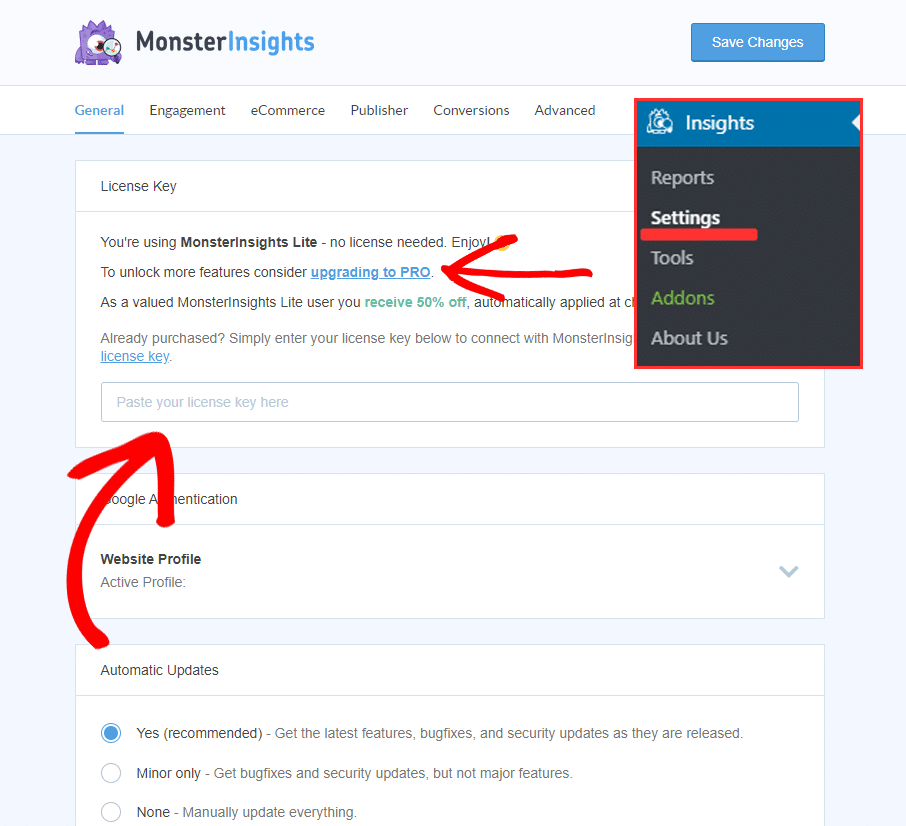This image is a detailed screenshot from the Monster Insights website, showcasing various interface elements and user edits. 

Starting from the top left, the image features the Monster Insights logo, characterized by a purple monster with a single eye holding a magnifying glass. To the right of the logo, the text "Monster Insights" is displayed, with "Monster" in dark blue and "Insights" in light blue.

On the top right, a blue button with slightly curved corners reads "Save Changes" in white letters. Below the top header, which has a light gray background, is the navigation bar. This bar has a white background and is bordered by thin gray lines above and below. The navigation options include: "General," "Engagement," "E-Commerce," "Publisher," "Conversions," and "Advanced." To the far right of the navigation bar is a blue button labeled "Insights," which acts as a dropdown menu. The dropdown menu is highlighted with a red outline drawn by the user and includes the options: "Reports," "Settings," "Tools," "Add-ons," and "About Us." The "Add-ons" option is marked in green, while the background of the dropdown is black, with most text in light gray except for "Settings," which is in white and underlined by the user.

In the main body content area, which has a light gray background, there are various sections with white backgrounds. The first section pertains to the license key, indicating that the user is using Monster Insights Lite with no licensing and suggesting an upgrade to Pro for additional features. The user has drawn an arrow pointing at "upgrading to Pro."

Further down in this section, there is a text field outlined in white, intended for pasting the license key. The placeholder text inside the box is in very light gray. Another red arrow, seemingly hand-drawn by the user, points to this field.

Below the license key section is a "Google Authentication" section, detailing options like "Website Profile" and "Active Profile." Following that is the "Automatic Updates" section, featuring three radio button options: "Yes, Recommended" for getting the latest features, bug fixes, and security updates; "Minor Only" for receiving only bug fixes and security updates without major new features; and "None" for manual updates.

These detailed elements and annotations by the user give a clear overview of the Monster Insights interface and specific areas of interest within the screenshot.